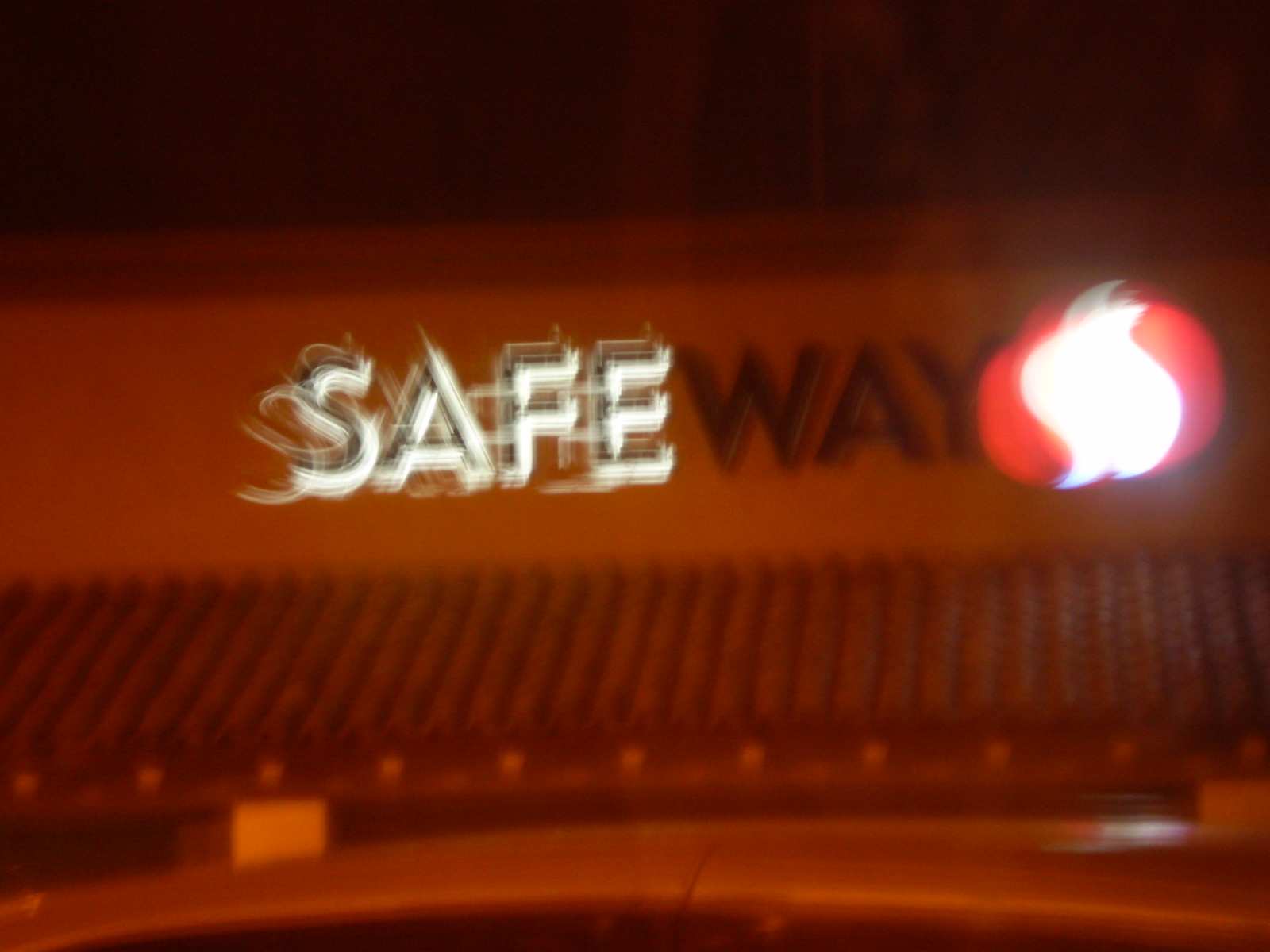This image captures the top section of a Safeway grocery store at night. The photo is notably blurry, contributing to the image's overall lack of sharp detail. Dominating the scene is an illuminated Safeway sign, with the word "Safe" appearing in white and "Way" in black, accompanied by the familiar red and white Safeway logo. Above the sign, the sky is dark, reinforcing the nighttime setting. Below the sign, a slanted, cobbled roof feature is visible, characterized by log-like shingles. Beneath this roofline, more of the store’s structure can be seen, and the blur in the image adds a glowing effect around the "Safe" part of the sign, which extends to the left. In the foreground, what appears to be the top of a car also comes into view, partially obscuring the lower portion of the store.